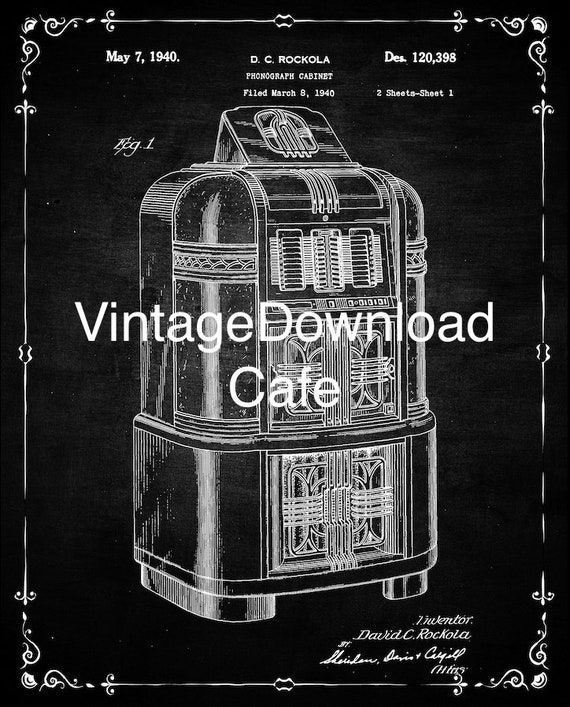A black and white poster prominently featuring a vintage jukebox-like machine at its center. The machine, intricately detailed with buttons and possible cabinet doors, is rendered in a white outline against a black background. Decorative patterns frame the entire image. In bold white letters near the middle, the text reads "Vintage Download Cafe." The poster includes several dates and text fragments: "May 7th, 1940," "DC Roccola," "Phonograph Cabinet filled March 8th, 1940," and "D.E. 120,398." Additionally, there is a cryptic notation: "December 120-398, Figure 1." This monochrome illustration offers a nostalgic glimpse into a bygone era.